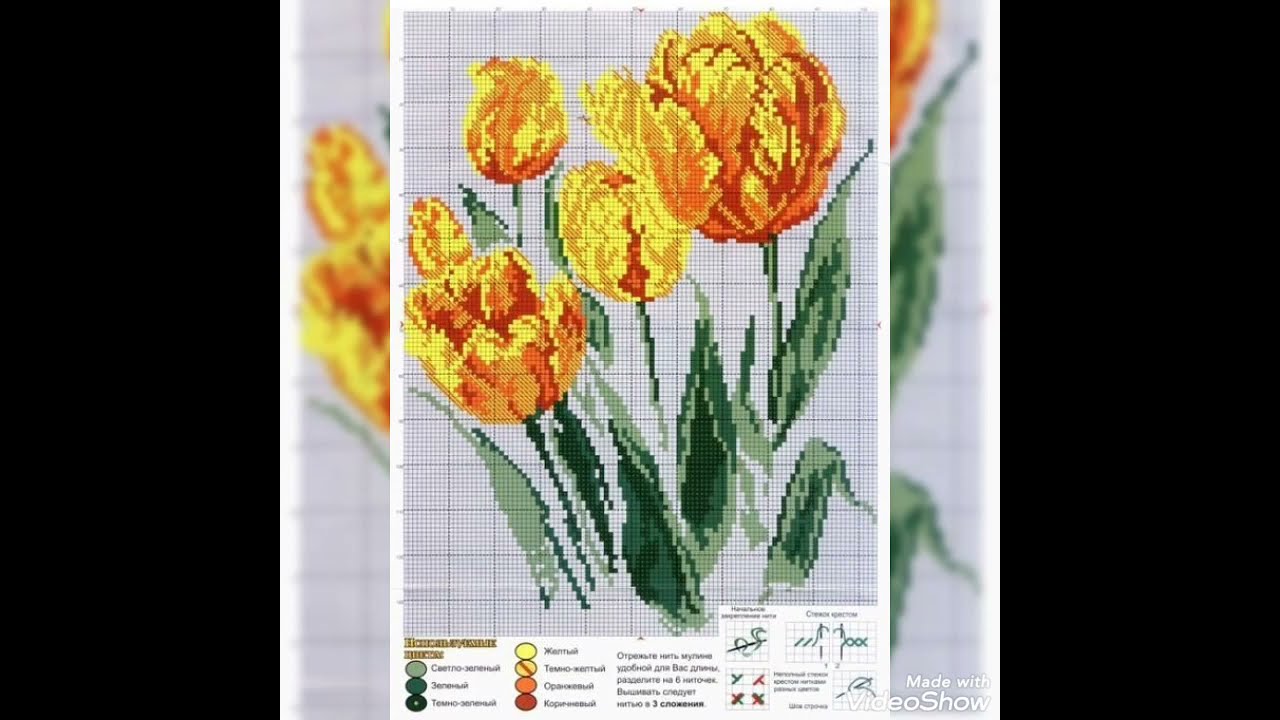This close-up photo captures a detailed pattern for a cross-stitch project. The main image showcases a cluster of tulips in yellow with orange highlights at their centers, arranged dynamically over a grayscale mat with measuring guidelines along the top and left edges. There are four distinct tulips: one large bloom on the right, another large bloom on the left, a smaller closed tulip in the back, and a central tulip just starting to open. Additionally, there appears to be a tulip bud tucked behind the lower left bloom. Surrounding these tulips are green stalks and leaves, accentuating the vibrant flowers. The lower portion features a comprehensive color guide, specifying the threads required, accompanied by detailed instructions and techniques for executing the cross-stitch, written in Russian. The image is flanked on the left and right sides by out-of-focus repeats of the central design, bordered further by black edges.